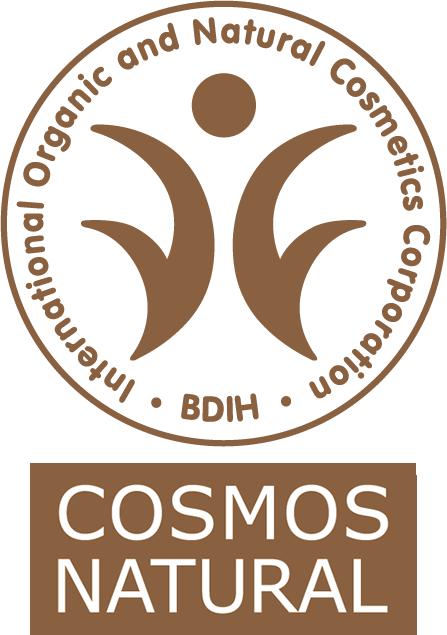The image displays a certification logo for the International Organic and Natural Cosmetics Corporation. Dominating the top portion, a brown circular emblem features the organization's name, "International Organic and Natural Cosmetics Corporation," inscribed along its inner rim. Flanked by dots, "BDIH" is prominently positioned at the bottom of the circle. Centered within this emblem, two brown leaf-like shapes mirror each other with a dot above them, resembling two outward-facing chicken feet. Below the circular emblem, a filled brown rectangle contains the label "COSMOS NATURAL" written in bold white capital letters, with "COSMOS" on the first line and "NATURAL" on the second. The logo, in entirety, employs a minimalist color scheme of brown and white, conveying an official stamp of approval for organic and natural cosmetic products.